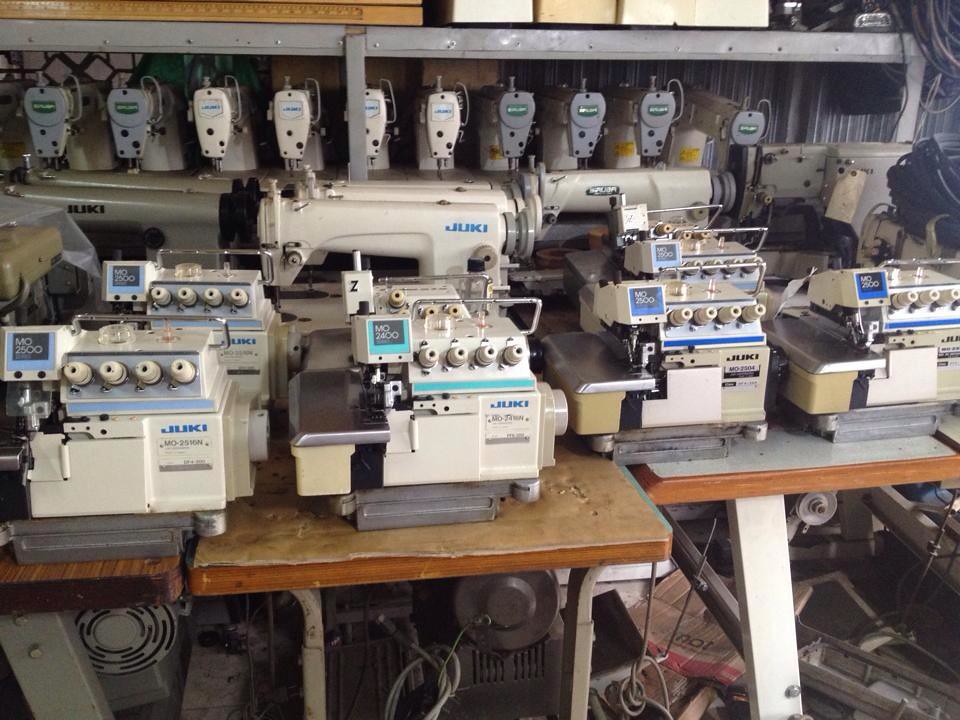The photograph depicts a cluttered workspace seemingly dedicated to the repair and manufacture of Juki (J-U-K-I) sewing machines. The room is densely packed with a variety of tables—some wooden, some white, and others makeshift with cardboard tops—and all are laden with numerous Juki sewing machines. Metal shelves along the walls are filled with additional machine parts and components, hinting at the complexity and volume of equipment in the space. The floor is scattered with miscellaneous scrap and parts, adding to the sense that this could be a back storeroom of a Juki repair shop or a factory setting. In the background, rows of more sewing machines and related equipment further contribute to the industrial atmosphere of this busy repair or production facility.